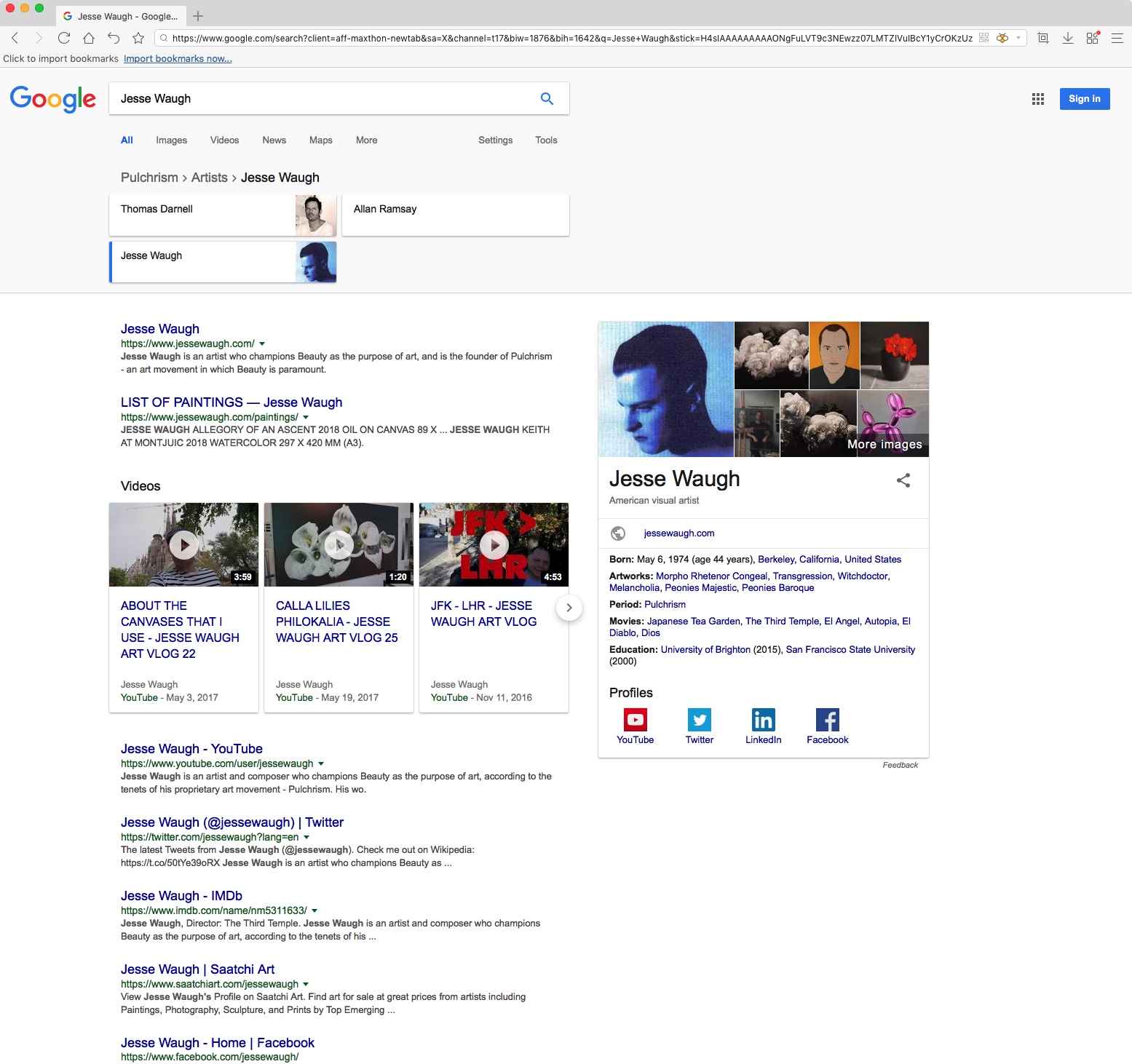Screenshot of Google Search Results for "Jesse Waugh"

The image captures a Google search results page in a web browser, with several distinguishable elements and intricate details:

1. **Browser Header**: 
   - The topmost section features a medium gray header.
   - At the far left, three colored circles appear in a sequence: a red circle, followed by a yellow circle, and finally a green circle.
   - To the right of these circles is a selected tab with a light gray background. It bears a multicolored 'G' logo on the left and is labeled with black text that reads "Jesse Waugh - Google...". 
   - Outside this tab, on top of the header, is a gray plus sign.

2. **Secondary Header Attached to the Tab**: 
   - Directly beneath the tab, the same color background extends to a secondary header.
   - This section features a left-pointing dark gray arrow, a right-pointing light gray arrow, and a refresh button.
   - Following these elements are the home button, back button, star button, and a white URL bar housing a light gray magnifying glass icon. Within the URL bar, there is an exceptionally long web address.
   - At the bottom left of this header, dark gray text reads "Click to import bookmarks," while to the right, blue underlined text says "Import bookmarks now...".

3. **Google Search Results Header**:
   - Below the secondary header is a light gray section for search results.
   - On the top left resides the iconic Google logo, illustrated with the letters "G," "O," "O," "G," "L," and "E" in blue, red, yellow, blue, green, and red respectively.
   - To the right of the logo is the search box, containing the black text "Jesse Waugh" on a white background. A blue magnifying glass icon is positioned on the far right of the search box.
   - Beneath the search box are multiple navigation options (All, Images, Videos, News, Maps, More) indicated in medium gray text, except "All," which is highlighted in blue, signifying it is the selected filter.
   - After some space appear additional options: "Settings" and "Tools," again in medium gray.

4. **Search Path and Results**:
   - Below this navigation bar, medium gray text shows "Pulchrism > Artists > Jesse Waugh," with "Jesse Waugh" bolded, indicating the current search path.
   - Following this line of text, the specific search results for "Jesse Waugh" are displayed, though the content of these results is not detailed in the description provided.